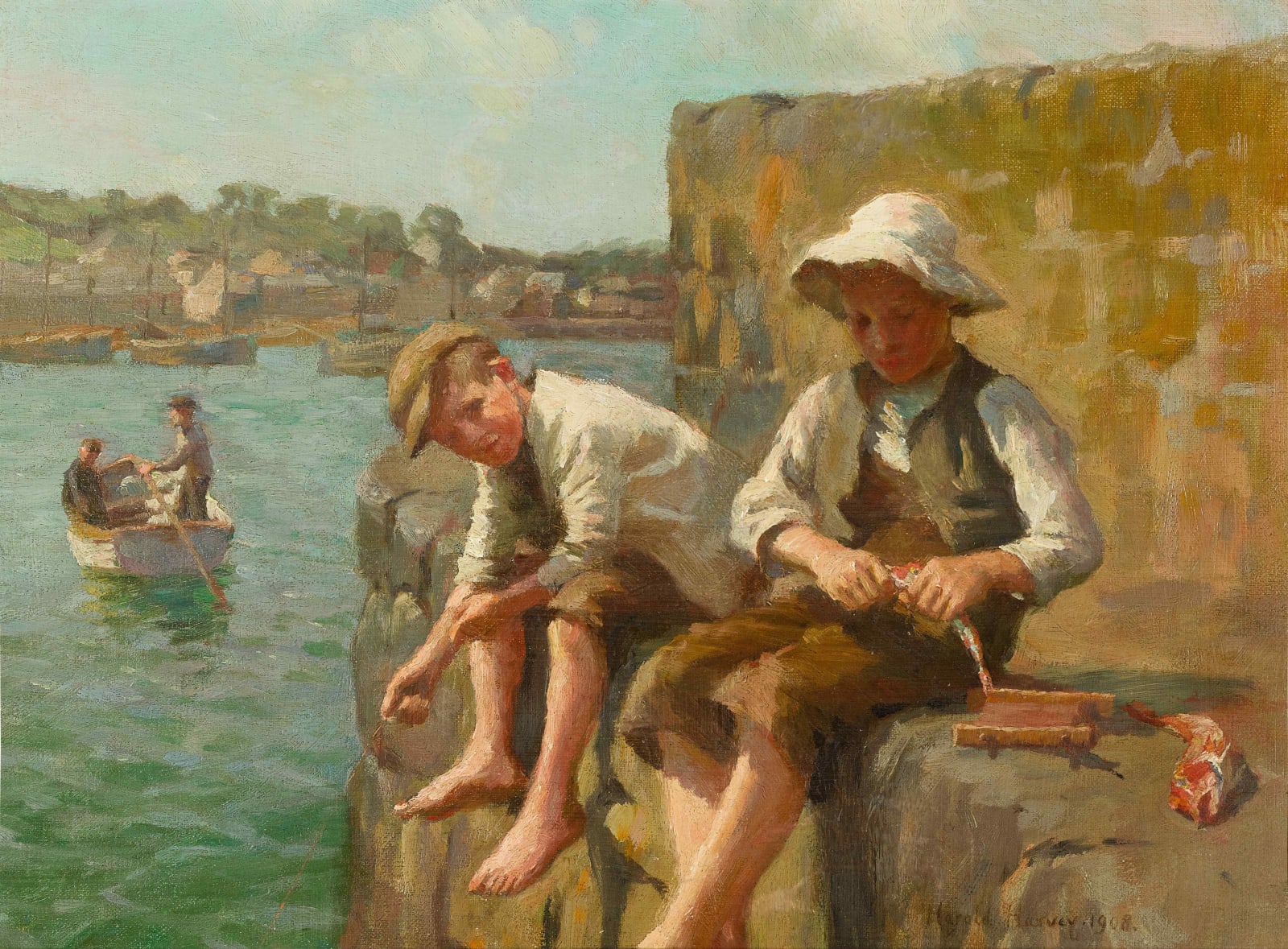This detailed watercolor painting, likely depicting a scene from the 1800s, captures a serene harbor. The calm blue-green waters are dotted with distant boats, including one rowboat with two men, one standing with a long paddle. In the foreground, two boys, reminiscent of Tom Sawyer, sit on a stone ledge. One appears disgruntled, facing the viewer, while the other is engaged with their catch, possibly filleting a fish. Both are in brown coveralls and white shirts, with one donning a flat cap and the other a fluffy sun hat. The muted colors and blurred clarity of the painting lend it a vintage, possibly European feel, evocative of the 1920s or 30s. A stone wall forms the backdrop of this tranquil riverside or lakeside scene.